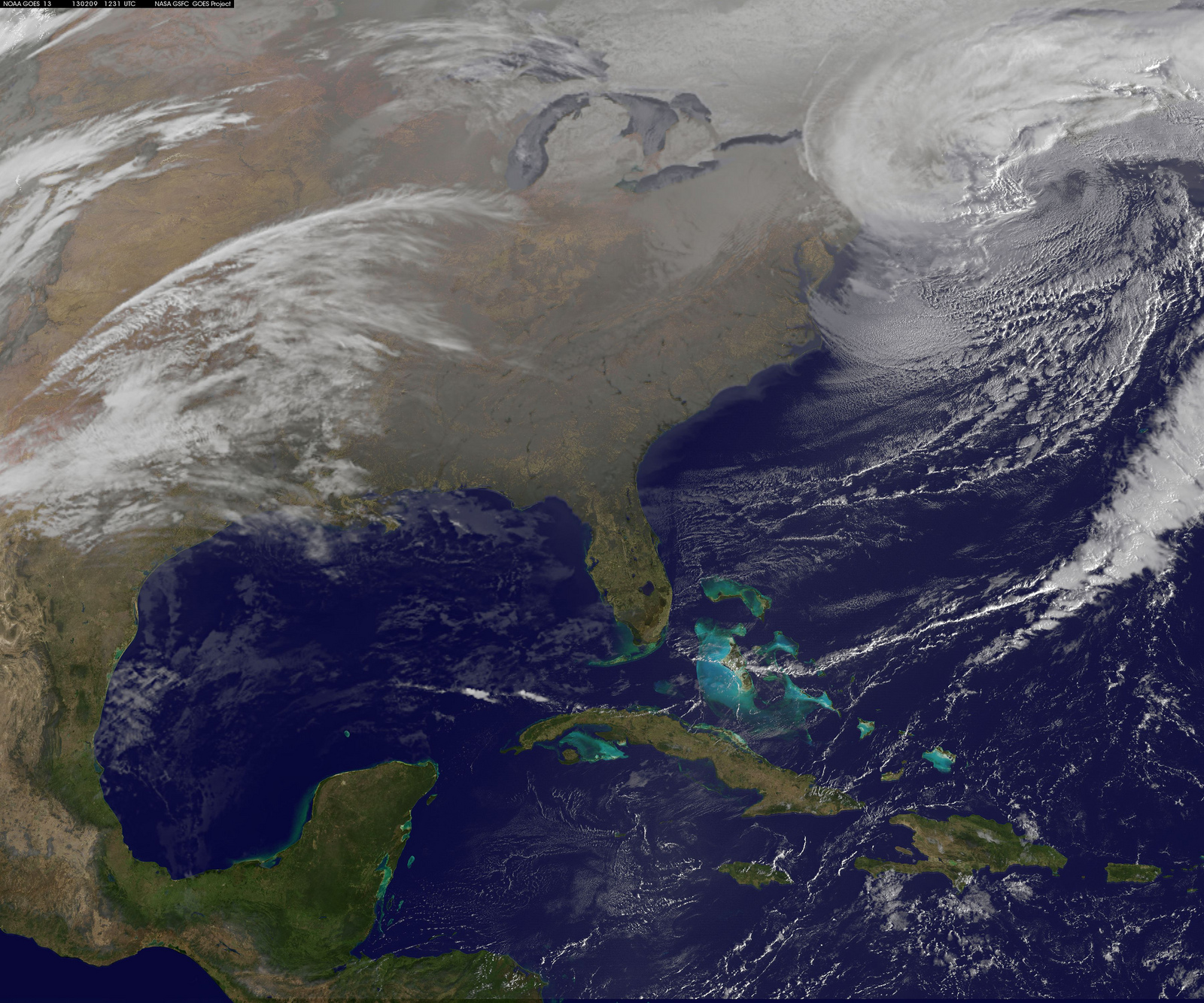This is a detailed satellite image taken from space, providing a sweeping view of the southeastern United States, primarily focusing on Florida and extending to parts of the Midwest, Mexico, and the Caribbean, including Cuba, Haiti, the Dominican Republic, Puerto Rico, and Jamaica. The northeastern part of the United States is heavily covered in clouds, rendering it almost unseeable, while the western and central regions display a drier, brown terrain. Florida and the surrounding islands are depicted with greener landscapes. The Gulf of Mexico and the ocean are shown in deep blue, almost purple hues, with noticeable green areas close to the Florida coastline, potentially indicating clearer waters or reefs. Swirling white clouds cover parts of the southern U.S. and the Caribbean region, contributing to the atmospheric texture. The image includes an unreadable tiny text box in the top left corner. Overall, the image combines vivid details of land, ocean, and cloud patterns as seen from space.